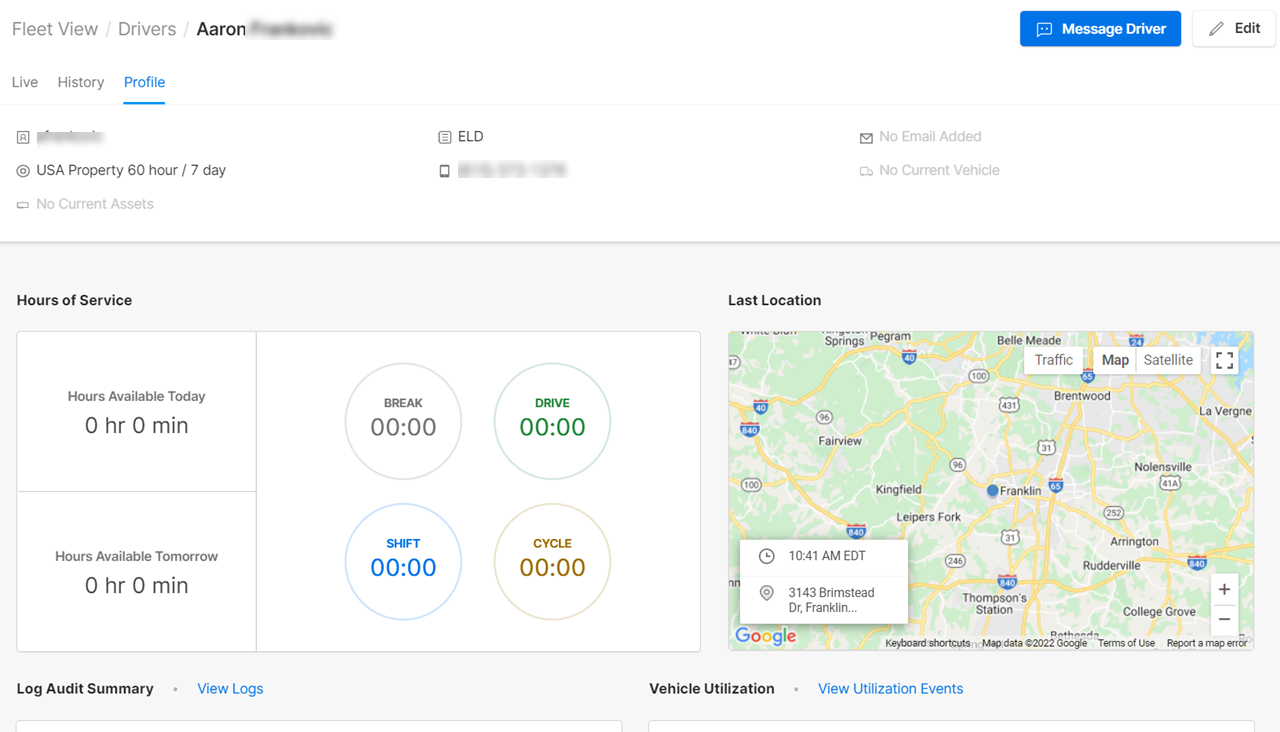The image displays a driving application interface, seemingly integrated with Google Maps. The top section is labeled "Fleet View," featuring various tabs such as "Drivers" and the driver's name, "Aaron," which is partially blurred out for privacy. 

There is an option in the upper right-hand corner to message the driver, currently highlighted in blue alongside an "Add" button. Additional tabs include "Live," "History," and "Profile," with "Profile" currently selected. The driver's name within the profile is also blurred. Fields for "ELD" (Electronic Logging Device) and "Email" are present, although it notes "No email added." 

The app indicates the driver is operating under USA property regulations, specifically the "60 hours/7 days" rule, with some relevant information blurred. It also states "No current vehicle" and "No current assets."

A horizontal light gray line marks a transition to a section titled "Hours of Service." This section contains two prominent fields: "Hours of Service" and "Last Location." Within "Hours of Service," details include:
- Hours available today: 0 hours, 0 minutes.
- Hours available tomorrow: 0 hours, 0 minutes.
Four status circles show times for various metrics:
- Brake: 0 hours (gray).
- Drive: 0 hours (green).
- Shift: 0 hours (blue).
- Cycle: 0 hours (yellow or brown).

Below this, users are prompted to log on to "Somerty.viewlogs." To the right, there's a map indicating the last known location of the driver, featuring standard map controls for traffic, satellite, etc. A time stamp reads "10:41 AM EDT" and it is pinned at "3143 Brimstead Dr, Franklin," though the location text is partially cut off.

The bottom section mentions "Vehicle Utilization" and "Utilization Events," though further detail is not visible in the image.